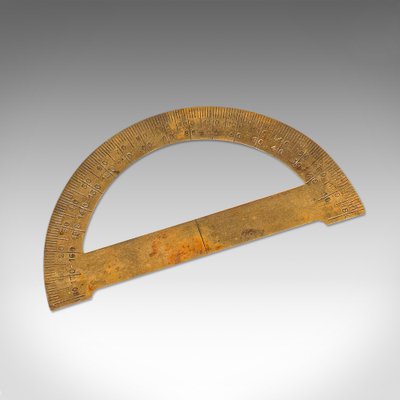The image features a metal protractor resting on a white surface, tilted diagonally with the right side elevated and the left side lowered. The protractor has a gold-colored finish, although it appears more likely to be made of another metal. The right bottom edge of the protractor is significantly darker, suggesting rust accumulation, while the left side also displays noticeable red rust spots. Despite the rust and wear, the etched numbers on the protractor’s surface are still visible, though they become blurred upon zooming in closely. The positioning of the protractor, with its inclined alignment, suggests it was deliberately turned to the side for this photograph.